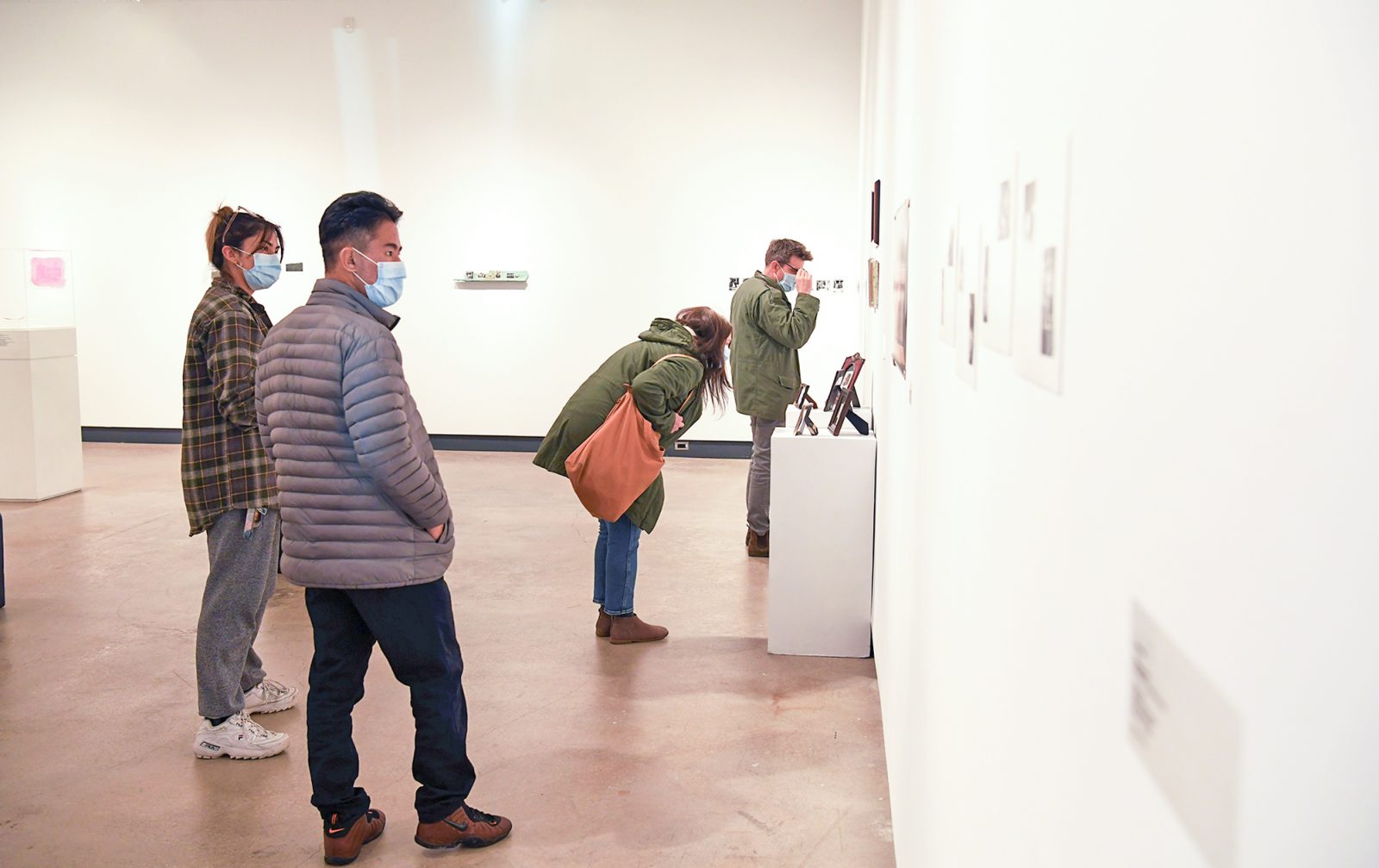In this detailed photograph inside a museum or art gallery, the setting features a room with a tan floor and stark white walls adorned with various paintings and photographs, some of which are mounted on stands. The image captures a diverse group of visitors, comprising two men and two women, all engaged with the art around them. 

In the foreground, an Asian man is seen in a gray parka, black pants, and brown shoes, his hands in his pockets while he looks downward at an image. He is wearing a blue face mask, indicative of COVID-19 precautions. Behind him, a white woman with brown hair, clad in a green plaid shirt, blue jeans, white sneakers, and also wearing a blue mask, stands attentively. She appears to be observing another piece of art or perhaps the same one the man is appreciating.

In front of them, a woman dressed in a green jacket with a large brown shoulder bag leans forward, scrutinizing framed images positioned on a stand. She has brown hair and is also in blue jeans and brown shoes, though her pink bag is distinct. Her face is turned away from the camera, making it unclear if she is wearing a mask. 

Further ahead, another man, white with glasses and a blue face mask, is absorbed in a painting on the wall. He is dressed in a green jacket and green pants. 

The room itself is lined with a black strip where the wall meets the floor, enhancing the room's minimalist aesthetic. Additional display cases and small objects are scattered throughout, contributing to the gallery's curated feel, though many are too distant to discern clearly.